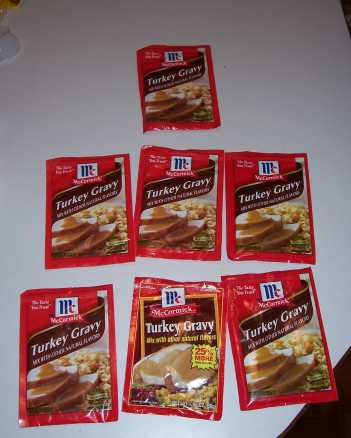A white countertop is scattered with multiple McCormick Turkey Gravy packets. Each packet prominently displays the McCormick logo, characterized by a blue 'M' and a red 'C'. The topmost packet features an image of succulent ham slices, drizzled with gravy, alongside what appears to be pasta. Below this packet is a neatly arranged row of three more McCormick Turkey Gravy packets. On the bottom left of the image, another Turkey Gravy packet is visible, mirrored on the bottom right. The packet in the center offers a slightly different design, showing the turkey slices more prominently toward the top left, revealing more of the dish underneath. This packet also includes additional graphics such as cranberries, stuffing, and a burst of yellow text highlighting a 25% promotion in a spiky yellow bubble.